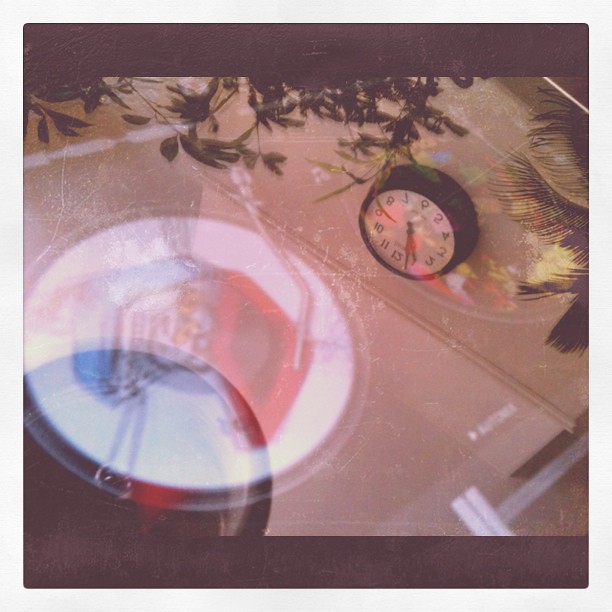This photo captures an intriguing reflection scene. The image is framed by a distinct brown border, enhancing the focus on the reflective elements within. At the center, there is a reflection of an indistinct object that features white, red, and blue colors, adding a sense of mystery. To the right, the reflection includes vivid details of surrounding greenery, notably showcasing a palm tree with its fronds splayed out. Additionally, the greenery includes another tree with green foliage, whose type is not immediately identifiable. Prominently featured is a black wall clock whose numbers and hands are clearly visible but appear upside down and reversed, contributing to the enigmatic nature of the reflection. The source of the reflection itself remains ambiguous, adding an element of curiosity to the image.